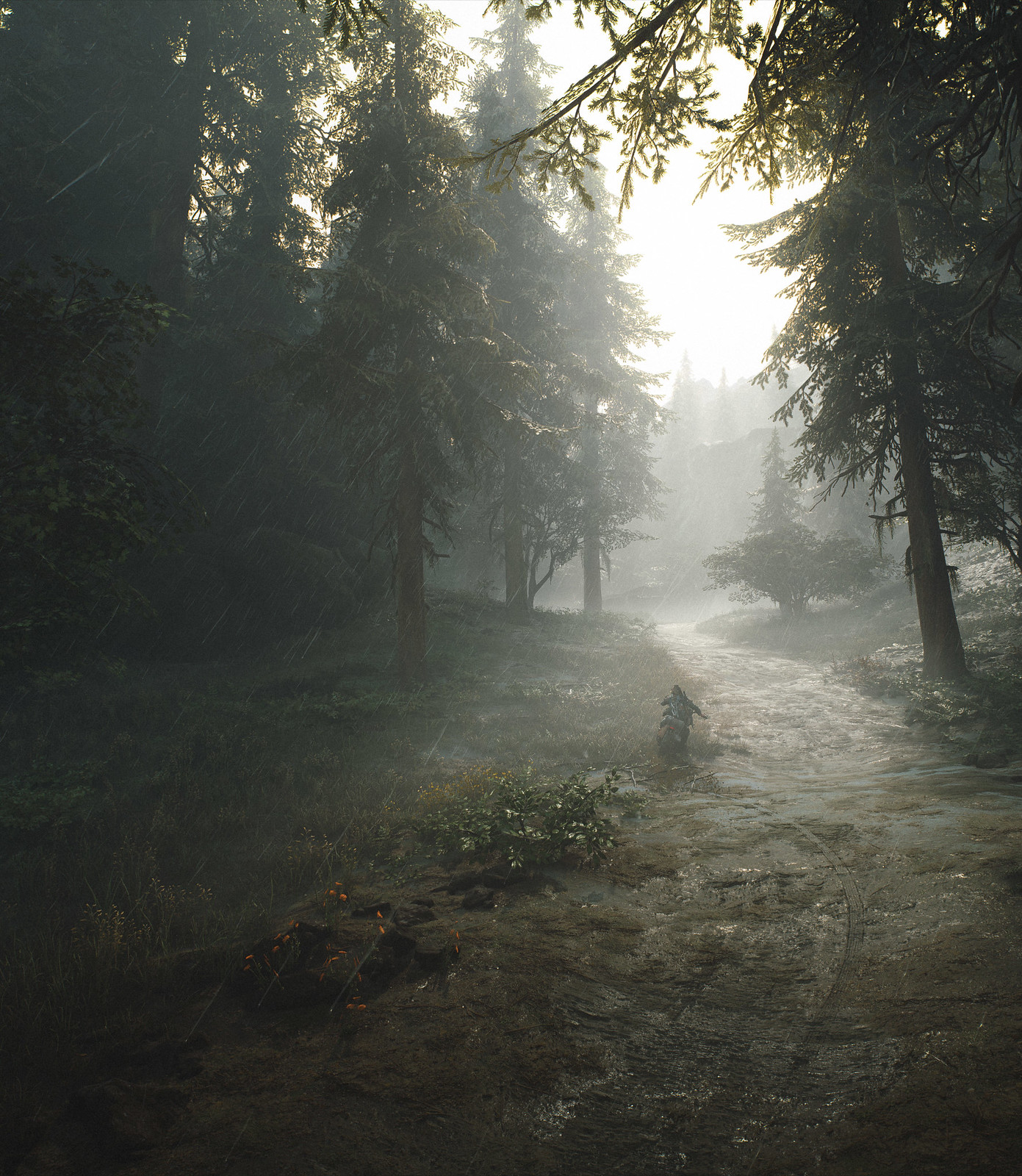This artwork, either a painting or digital illustration, captures a serene landscape featuring a misty forest with numerous spruce and evergreen trees. The composition is dominated by a bright sun positioned in the center upper-right section, casting a luminous, white light that bathes the entire scene. This radiant sunlight contrasts vividly with the shadowy lower corners of the image. A worn path winds its way through the foreground, leading the viewer’s eye deeper into the forest, where the dark green evergreens stand tall and majestic. To the lower left, a small grassy opening adds a touch of verdant detail, enhancing the natural beauty of the scene. The overall mood is one of tranquil solitude, inviting the viewer to lose themselves in the peaceful embrace of the forest.